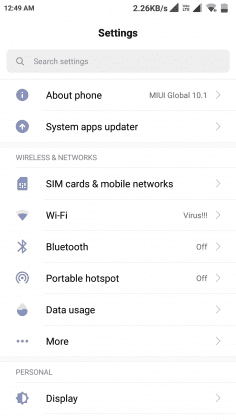The image is a screenshot of a cell phone screen captured at 12:49 a.m., as indicated by the clock in the upper right-hand corner. The screenshot showcases several on-screen elements, including a data download rate of 2.26 kilobytes per second, multiple cellular signal strength indicators, an LTE icon, a Wi-Fi icon, and a battery icon showing roughly 25% charge.

The background of the screen is predominantly white. At the top, the word "Settings" is prominently displayed above a search bar labeled "Search settings." Below the search bar, several menu options are listed, beginning with "About phone," followed by "MIUI Global 10.1" and "System apps updater."

The next section is categorized under "Wireless networks," with subsections such as "SIM cards and mobile networks," "Wi-Fi," and a striking entry labeled "Virus!!!" with three exclamation points, which stands out among the otherwise typical settings options. Further down the menu, "Bluetooth" is labeled as "Off," "Portable hotspot" is marked as "Off," and there is a "Data usage" section followed by a set of three dots indicating additional options. The last listed item in the screenshot is "Display."

Each of these menu items features a right-facing arrow on the right-hand side, suggesting that clicking on them will expand to reveal more options. Additionally, a light blue emoji is positioned to the left of each setting, adding a touch of color to the otherwise minimalistic design.